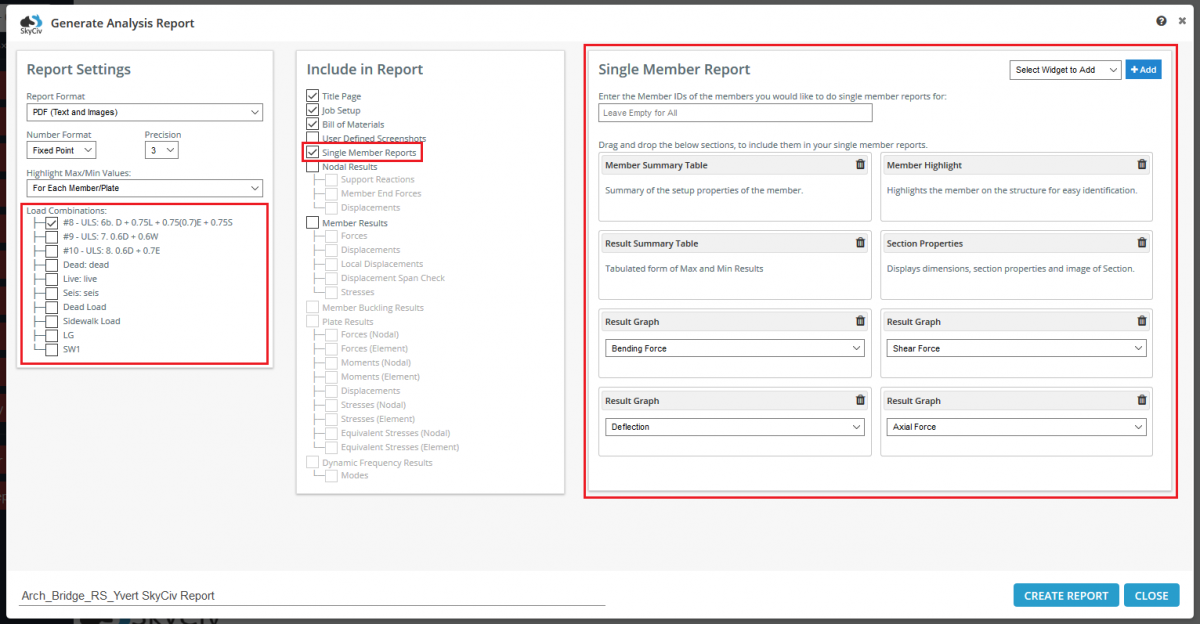This detailed image shows a user interface for generating an analysis report. The top left corner features the title "Generate Analysis Report." Directly below, there are various configuration settings including "Report Settings," with options for "Report Format," where PDF, Text, and Images are selectable formats. The "Number Format" is set to fixed point, and the "Precision" is configured to 3 decimal places. Additionally, there is an option to "Highlight Max Min Values," and for each member, the "Each Member Plate" option is chosen.

In the middle of the interface, there's a section titled "Include in Report," with checkboxes for different items: "Title Page," "Job Setup," "Bill of Materials," and "Single Member Reports." The "Single Member Reports" option is not only checked but also highlighted with a red box for emphasis.

To the right, a large red box encloses a significant amount of detailed instructions. The top of this section is labeled "Single Member Report," with a prompt to "Enter the member IDs of the members you would like to do Single Member Reports for." A text box is provided, indicating "Leave Empty for All" as an option. Further below, there are instructions to "Drag and Drop the below sections to include them in your Single Member Reports."

The categories available for inclusion are:
1. **Member Summary Table** - A summary of the setup properties for each member.
2. **Member Highlight** - Highlights the member on the structure for easy identification.
3. **Result Summary Table** - Provides a tabulated form of the maximum and minimum results.
4. **Section Properties** - Displays dimensions and section properties.
5. **Image of Section** - Visual representation of the section.

Additionally, there are multiple "Result Graph" options, each with a pull-down menu offering choices such as "Bending Force," "Shear Force," "Deflection," and "Axial Force." This comprehensive setup allows users to fully customize the content and format of their generated analysis report.